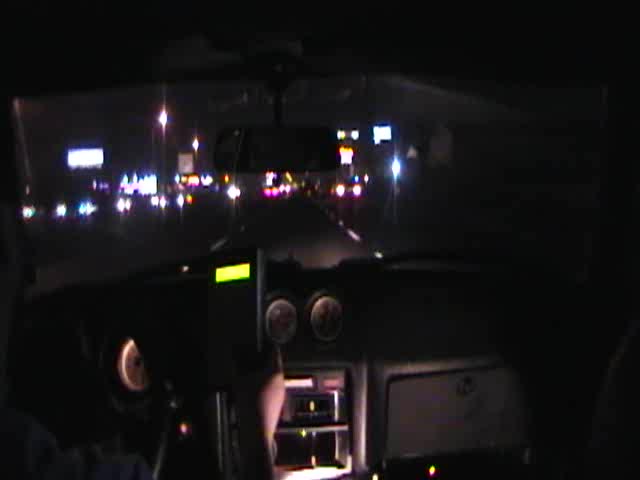The image is a detailed photograph taken from inside a vehicle during the evening. From within the car, almost the entire dashboard is visible, including the glove compartment, radio, and steering wheel. One arm is seen resting on the steering wheel. The rearview mirror is also in view, along with the windshield and windshield wipers. Outside the vehicle, the road stretches ahead, demarcated by white lines on both sides. In the distance, the headlights and taillights of other cars travel in both directions. Business signs dot the sides of the road, and a stoplight is prominently visible in the foreground. The car’s interior remains mostly dark, except for the illuminated gauges on the dashboard displaying information like the speedometer.